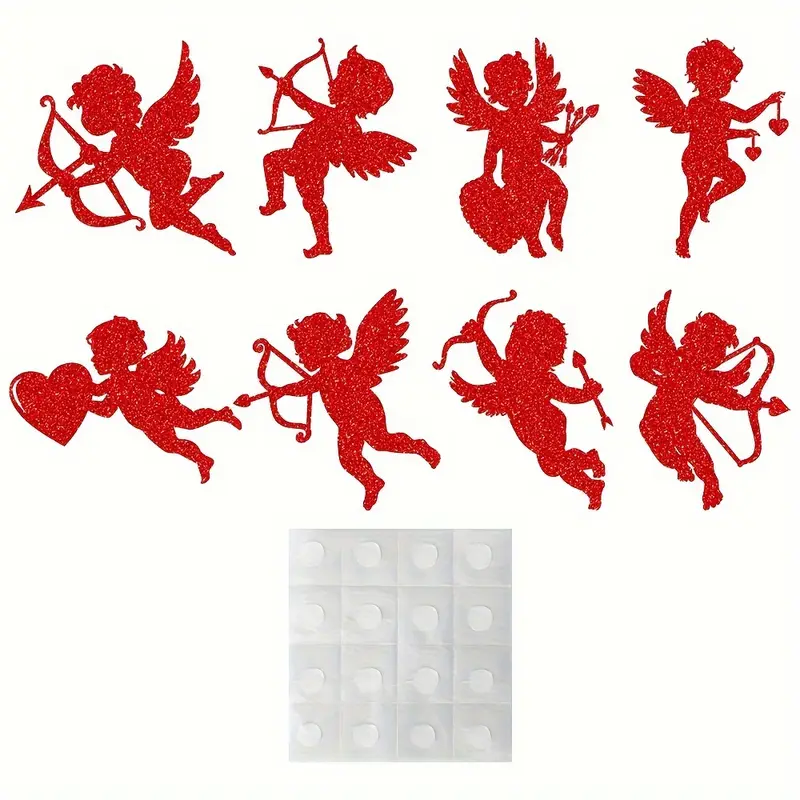This image features a collection of eight detailed red silhouettes of Cupid in various dynamic poses, all arranged neatly within a two-by-four grid on a stark white background. Each Cupid figure stands out in minimalistic red, highlighted by the intricate outlines of baby-like forms complete with wings, bows, and arrows. The top row displays one Cupid in a side profile aiming a bow and arrow, another with an arrow pointed upward while balancing on one foot, a third facing forward with wings spread wide, holding a bunch of arrows and a heart, and a fourth clutching two hearts dangling from its hands. The bottom row showcases a Cupid holding a giant heart, another aiming an arrow downward, a third with a bow in one hand and an arrow in the other, and the last pointing right as it shoots a bow and arrow. Below this colorful display, there is a white piece of paper divided into 16 quadrants, likely created by folding and unfolding it multiple times, with a white dot in the center of each square, possibly made from glue or paint.